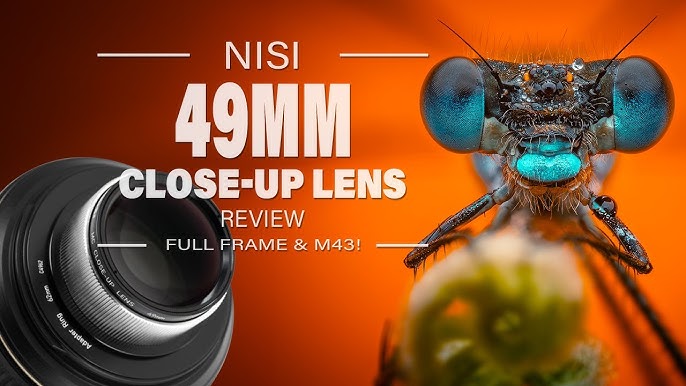The image is a detailed advertisement for a NISI 49mm close-up camera lens, prominently featuring an orange background. The left side of the rectangular layout includes a black camera lens positioned at a 45-degree angle, revealing part of its optical interior. The text, written in white, reads "NISI," followed by "49mm," "Close-Up Lens Review," "Full Frame," and “M43!” On the right side of the image, there’s a highly detailed macro photograph of a black insect, likely a fly, showcasing its striking blue eyes and blue-tinted facial features. The fly’s head is in sharp focus, with its hairy legs and slightly blurred body giving a sense of depth and precision achievable with the advertised lens. The composition effectively highlights the lens's capability for extreme close-up photography.